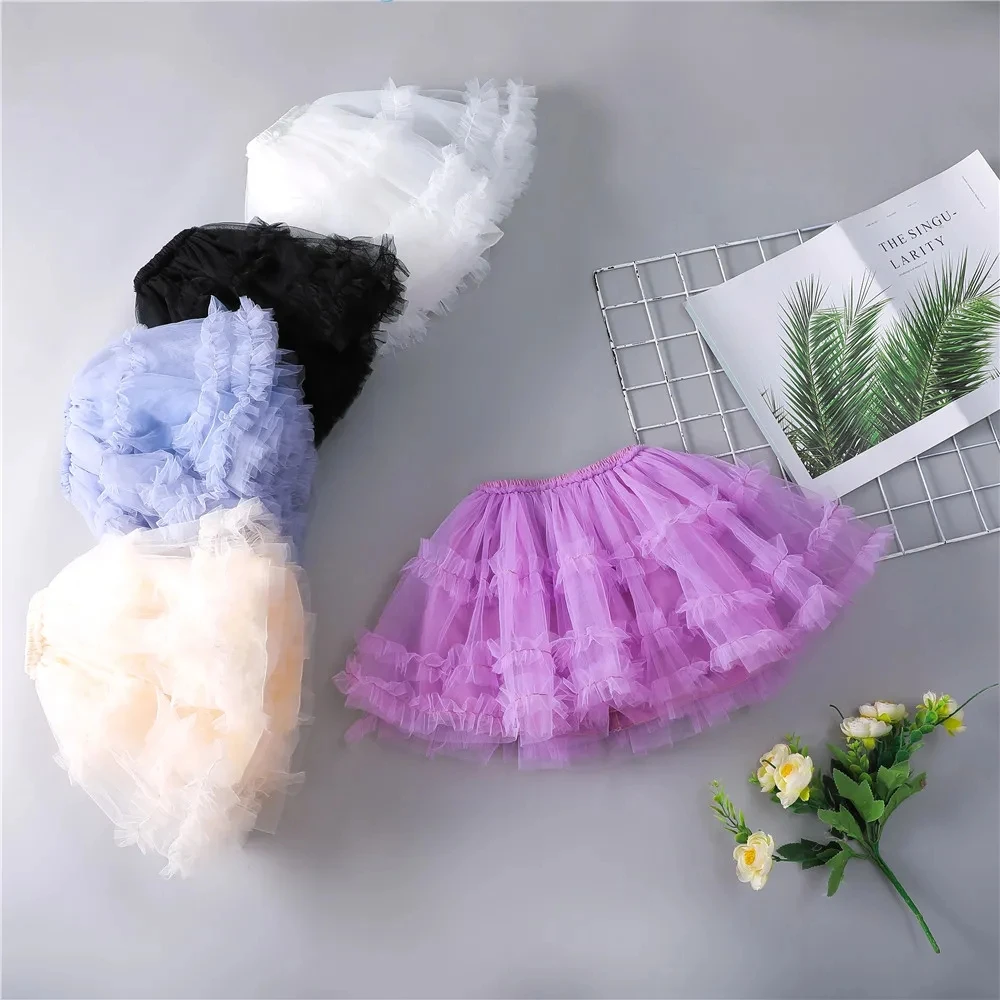The image is a highly detailed and artistic setup, possibly meant for an Instagram photo. Dominated by a visually complex arrangement, the centerpiece features a series of ballerina tutus arranged diagonally from the lower left to the upper right. The tutus are layered in a sequence: the first is cream-colored, followed by light blue, black, and then white. To the right of this row, there is a flat, lavender-colored tutu, all seemingly of the same tulle design with silver mesh underneath.

Adding to the aesthetic complexity, the background is a stark gray which contrasts with the vibrant colors of the tutus. The setup includes a metallic grate, possibly once white but now peeling, adding a textured grid beneath the arrangement. Resting on this grate is an open booklet titled "The Singularity," adorned with images of leaves on a white background. The paper appears to be well-used, showing folds and creases. 

In the bottom right-hand corner of the image, there is a delicate stem of white and yellow flowers with green leaves, subtly complementing the color scheme. Below the lavender tutu, a bouquet of what appears to be artificial flowers adds to the picturesque quality of the setup, evoking a theme that could be hinting at a dance recital or an elegant display of ballet costumes.